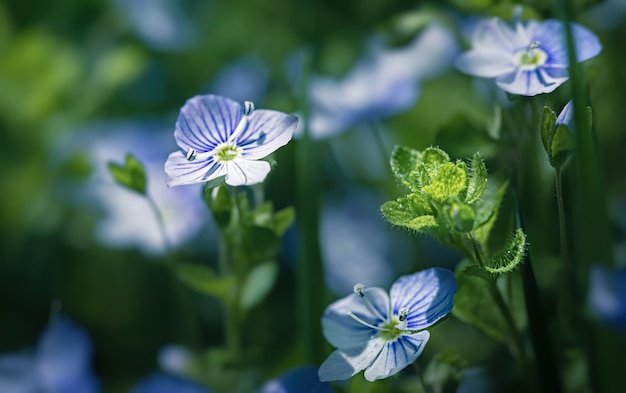This captivating close-up photograph showcases three richly detailed flowers in sharp focus, standing out against a softly blurred background of similar blooms. Each flower features four delicate petals with striking blue streaks emanating from a greenish center, creating a vivid visual contrast. The centers of the flowers reveal small green circles and two protruding pollen spikes. Encircling these blooms are fuzzy green leaves that add to the intricate texture of the image. To the right, there is an unbloomed flower bud with curved-up leaves, covered in tiny hairs, hinting at its impending bloom.